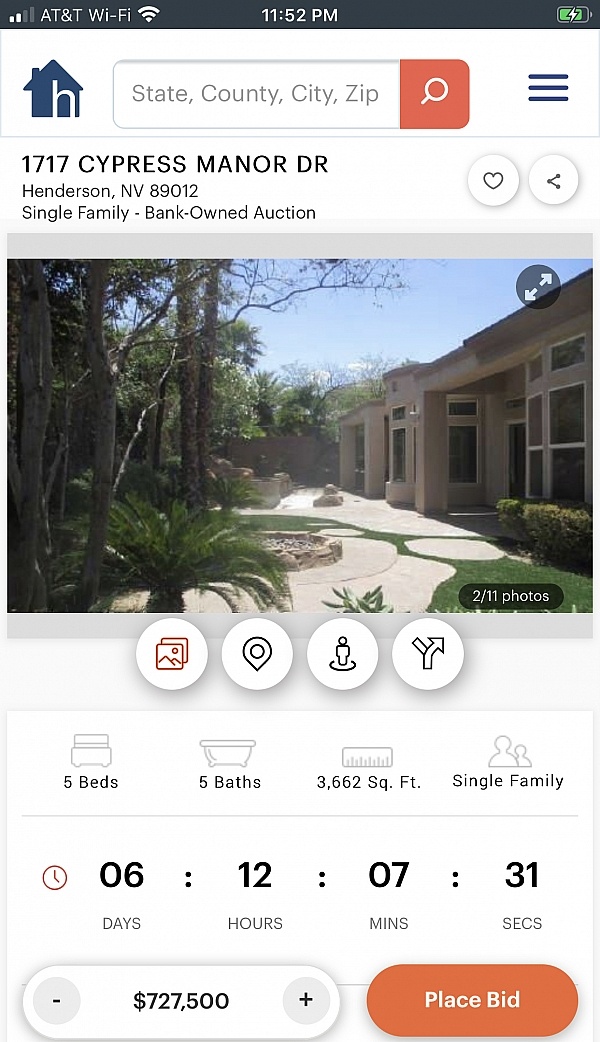Screenshot of the Homes.com App Interface

The screenshot captures the Homes.com mobile app interface. At the top left corner, a blue house with an "H" inside represents the Homes.com logo. To its right is a search bar, and further right, a red box featuring a white magnifying glass icon. On the far right, there's a three-line menu icon.

Below this header, in bold print, is an address. Centered beneath it are the street details and city information. At the bottom of this section, the property is labeled as a "Single Family Bank Owned Auction." Next to it, options for "hearting" (favoriting), liking, or sharing the property are provided.

Dominating the center of the screenshot is a large photo of the house's front exterior. In its top right corner, a black circle with diagonal arrows allows users to maximize or minimize the photo. At the bottom right, text indicates "2 out of 11 photos." Along the bottom edge of the photo, four icons are aligned: one for photos, another for location, a third for adjusting the view, and a fourth for directions.

The bottom section of the screenshot features five icons with information: a bed icon with "5 Beds," a bathtub icon with "5 Baths," a ruler indicating the square footage, and people icons signifying "Single Family." Additionally, a timer displays "6 days, 12 hours, 7 minutes, 31 seconds left in the auction." On the bottom left is a numeric box for adjusting the bid, and to its right, an orange button labeled "Place Bid."